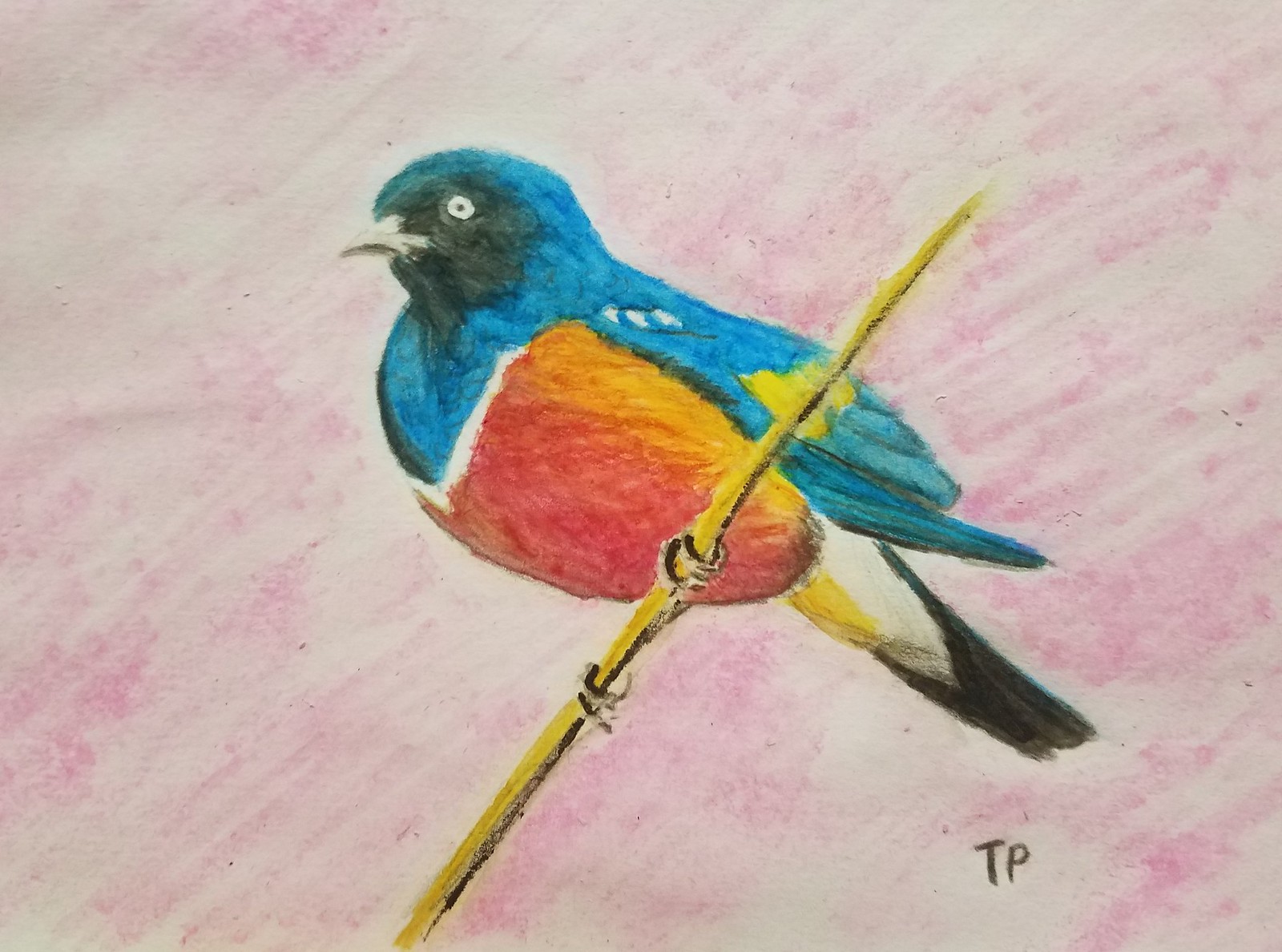In this captivating watercolor or colored pencil drawing, a vibrant bird is perched gracefully. The bird's lower belly is richly colored in red, complemented by a striking blue section. It stands on a yellow branch, its feet firmly grasping the perch. To the right, the artist has intriguingly included the initials "teepee" as part of the composition. The top left corner of the image features a prominent white eyeball with a single dot, adding a whimsical element to the artwork. The background is a soothing blend of pink and white hues, providing a gentle backdrop that makes the bird's colors pop. The artist's signature, "R," followed by "teepee," is neatly inscribed, completing this detailed and imaginative piece.